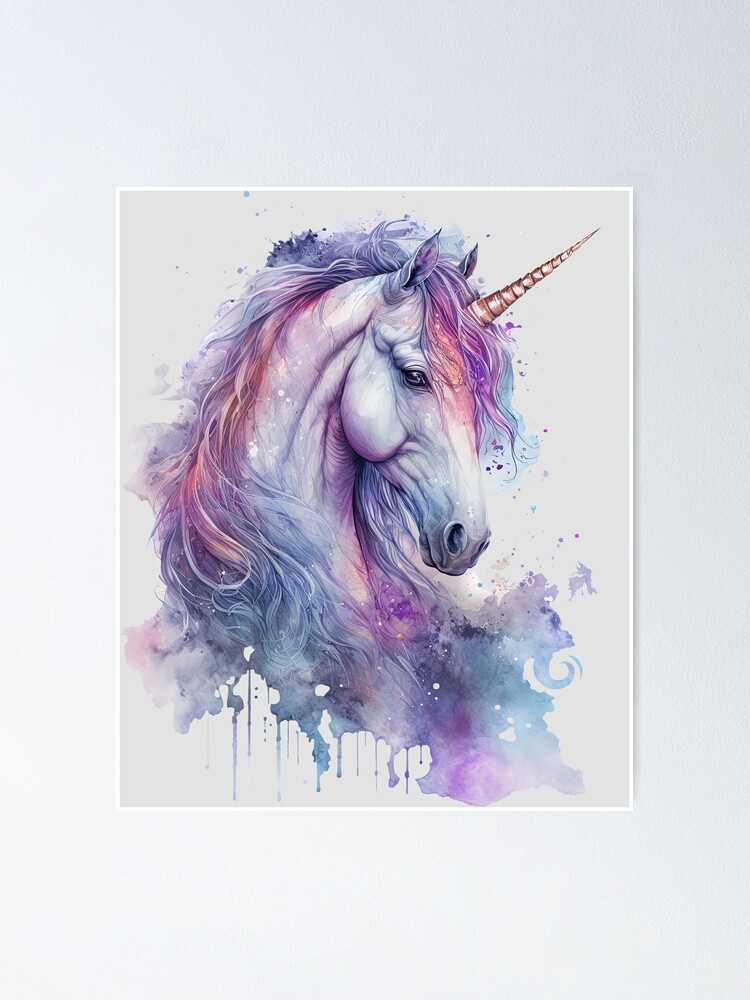The image depicts a detailed watercolor painting of a unicorn mounted on a light gray wall, enclosed within a thin white border. The painting itself is vertically oriented, capturing the unicorn from the neck up and facing to the right. The unicorn's skin is a delicate blend of white with subtle hints of purplish-gray, and it has dark black eyes. A prominent gold horn emerges from its forehead, surrounded by soft touches of pastel pinks and oranges. The unicorn's mane is an intricate cascade of pastel purples, grays, pinks, and oranges, flowing from around the horn to just above its nose, and then down its neck. The mane gradually transitions into colorful paint blobs and watercolor drips, forming a rainbow-esque cloud at the bottom of the image. The painting showcases the lumpy, ridged texture of the unicorn's face, enhancing the watercolor effect with its dripping appearance.